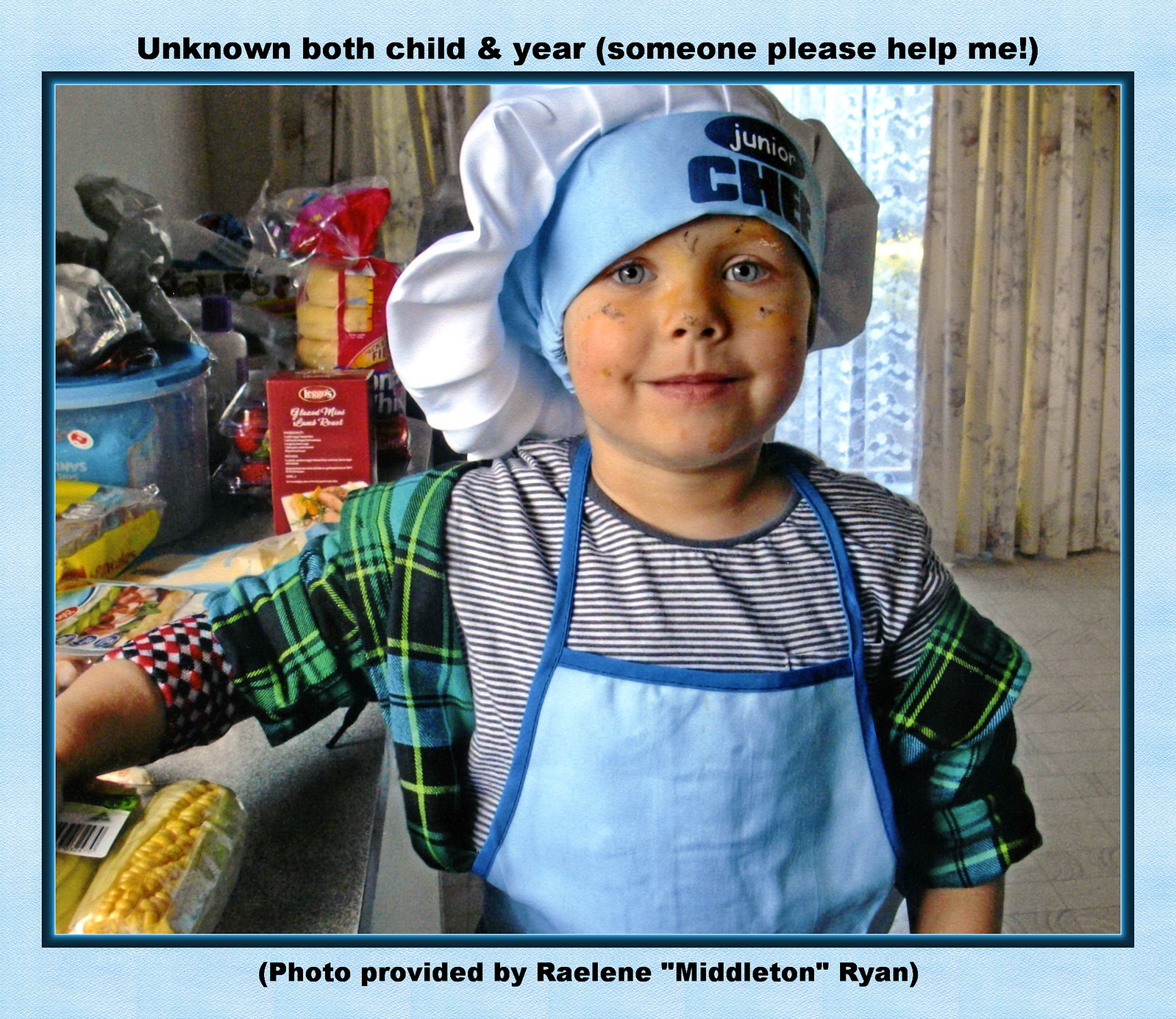The photograph shows a young boy, approximately four years old, standing slightly right of center and facing the viewer. He is dressed as a chef, wearing a blue apron over a striped bib and a green and black plaid shirt, with a blue and white "Chef Junior" hat perched atop his head. His face is dirty, and he has striking blue eyes. The boy's right arm rests on a countertop filled with various food items, including mixes, bagels, and packaged corn. Behind him, the living room is visible with its draperies and rug. The image is placed within a solid light blue rectangular background, with a caption at the top in black text that reads, "Unknown, both child and year. Someone please help me!" and a bottom caption that states, "Photo provided by Raylene Middleton Ryan." The style of the photograph combines representationalism with typographic elements.